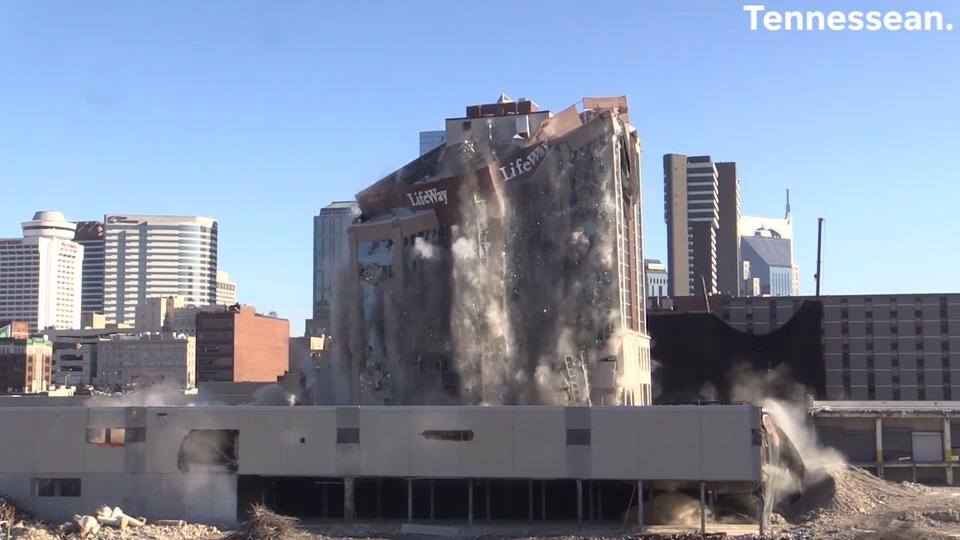In this daytime color photograph, a building labeled "LifeWay" is captured in the midst of a dramatic collapse, likely a controlled demolition. The building is disintegrating into rubble and dust, creating a smoky atmosphere around it. In the foreground, a parking garage is partially visible, covered in debris. The city skyline forms the backdrop, featuring various office buildings and skyscrapers under a clear blue sky. The image is marked in the top right corner with the watermark "Tennessean."